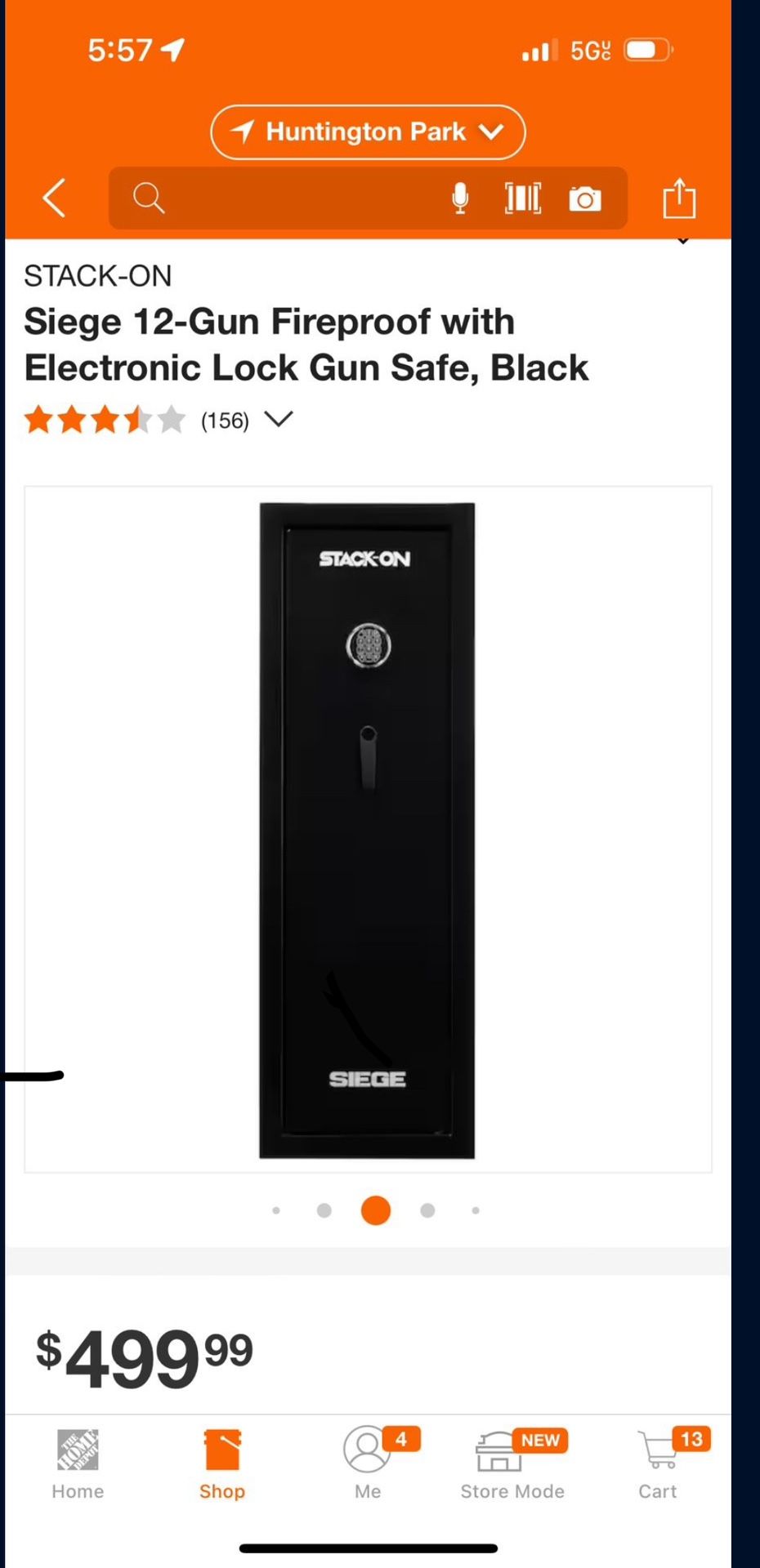The image depicts a smartphone screen displaying a product page from The Home Depot website. At the top of the screen, there is an orange strip with the number "557" on the left and various status icons on the right, including a bar indicator for cellular signal strength, a "5G" symbol, and a battery indicator.

In the middle of the screen, "Huntington Park" is displayed within an oval. Below that, there is a left-facing arrow on the left, a search bar in the center, and an upload icon on the right.

The main content shows a product, specifically a Stack-On S12GUN Fireproof Gun Safe with an electronic lock, colored black. The product has a 3.5-star rating based on 156 reviews. There is a pull-down menu available for additional options.

The gun safe has five photos displayed at the bottom, with the middle one being highlighted in orange while the others are gray. The price of the product is listed as $499.99.

At the bottom of the screen, navigation options are indicated - "Home" is currently selected. Adjacent to it are "Shop," "Store Mode" (marked as new), and "Cart," which shows 13 items with an orange rectangle and the number 13 in white.

Overall, the screen has a white background and focuses on the featured gun safe product available for purchase at Home Depot.